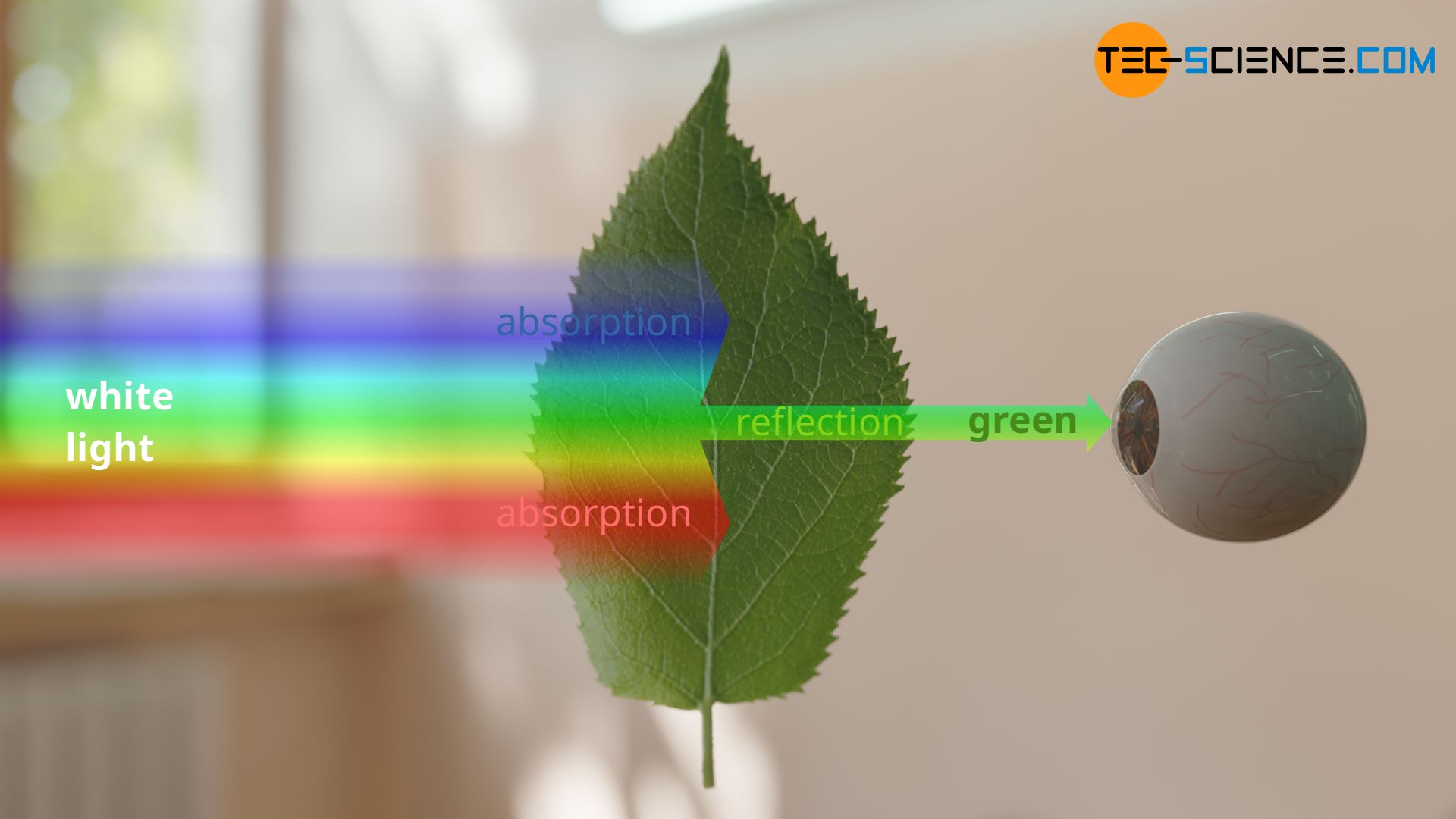The image features a vertically positioned, narrow green leaf at the center, set against a white background suggestive of an office or home setting. To the left of the leaf, a spectrum of colors—blue, green, yellow, orange, and red—illustrates the various wavelengths of light. Text labels near the blue and red sections indicate that these colors are absorbed by the leaf, while a "white light" label is situated centrally. On the right side, the green color is marked as being reflected. Accompanying this setup is a detailed depiction of a human eye with a brown iris and visible blood vessels, connected to the leaf by an arrow signifying the process of color perception. The top right corner bears the label "tech-science.com," indicating the source of the diagram. The image overall visually explains how light absorption and reflection determine the green appearance of the leaf as interpreted by the human eye.